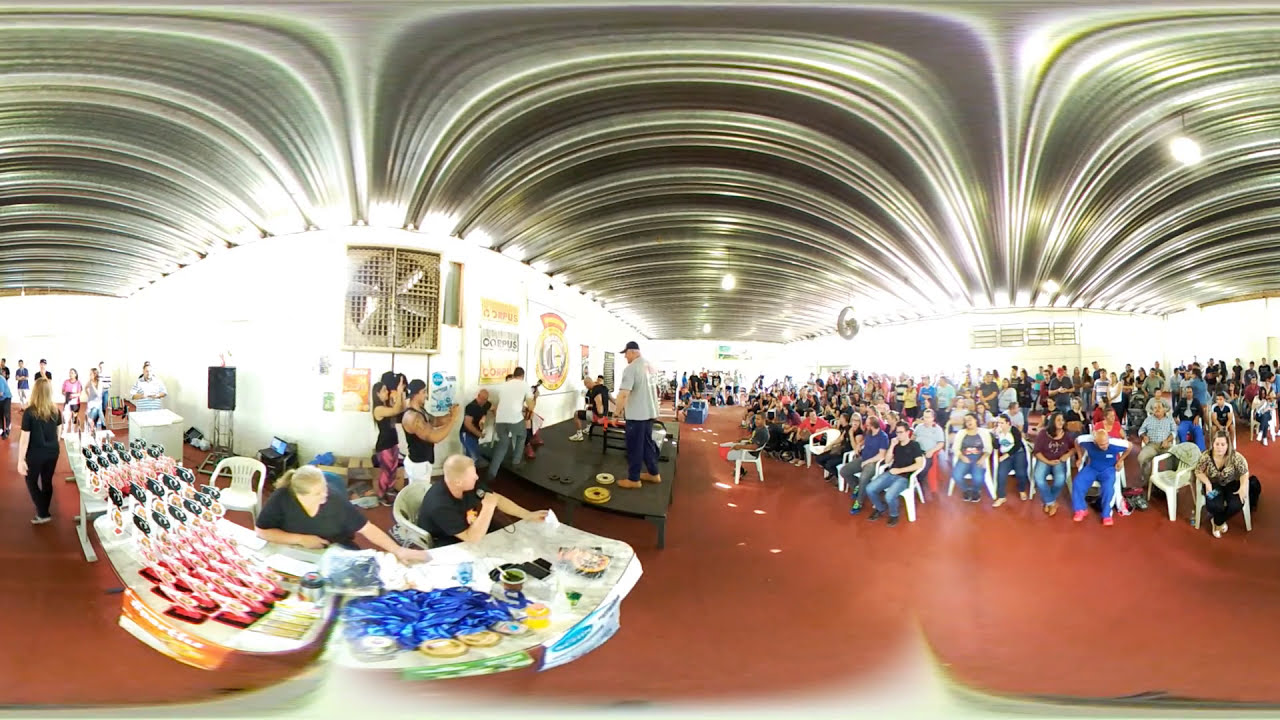The image depicts a 360-degree view of a large room with white walls and an arched metal roof, possibly a convention or event space. The floor is red, and industrial fans are visible on the walls. In the middle of the room, there's a low black stage with some weights on the ground, indicating a weightlifting competition or demonstration. A person holding a microphone appears to be talking about the event happening on stage.

In the foreground and extending towards the back left, there is a long table covered with various snacks and items, possibly for sale. People are manning these tables, and a couple of them are in black shirts and seated in white plastic chairs. Several individuals with cameras are positioned behind the tables, pointing towards the stage to capture the event.

On the right-hand side, a large audience is seated in rows of white plastic chairs, attentively watching the stage. The audience members are dressed casually in blue jeans, t-shirts, khakis, and light sweaters. The room is well-lit, giving a clear view of the entire setup, including the stage, tables, and audience.